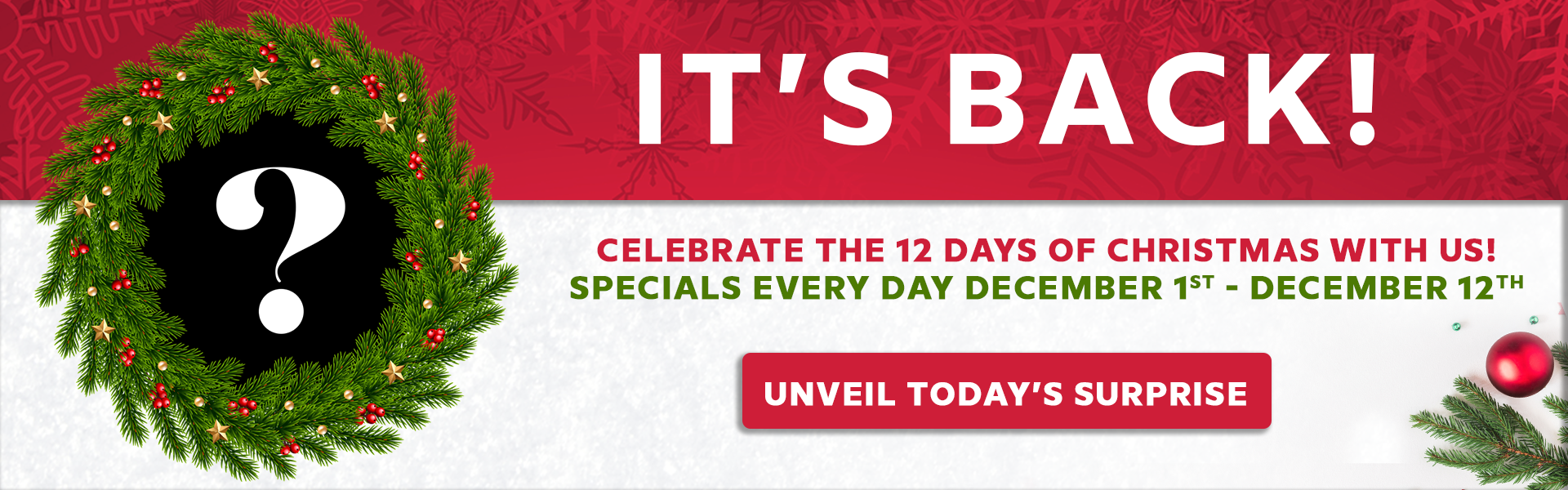In this small rectangular online advertisement, the left side prominently features a lush green spruce wreath adorned with small red berries, light tan pearl-like objects, and brass or copper stars for decoration. At the center of the wreath, a black background showcases a large, bulky white question mark. To the right, the text "It's Back" is displayed in bold white font against a red background adorned with darker red snowflake patterns. Below this, the phrase "Celebrate the 12 Days of Christmas With Us" is written in red, followed by "Specials Every Day December 1st through December 12th" in green. At the bottom, a red rectangular button with white text reads "Unveil Today's Surprise." In the bottom right corner, a bushy spruce branch is visible, accompanied by a red berry or bauble ornament just above it.